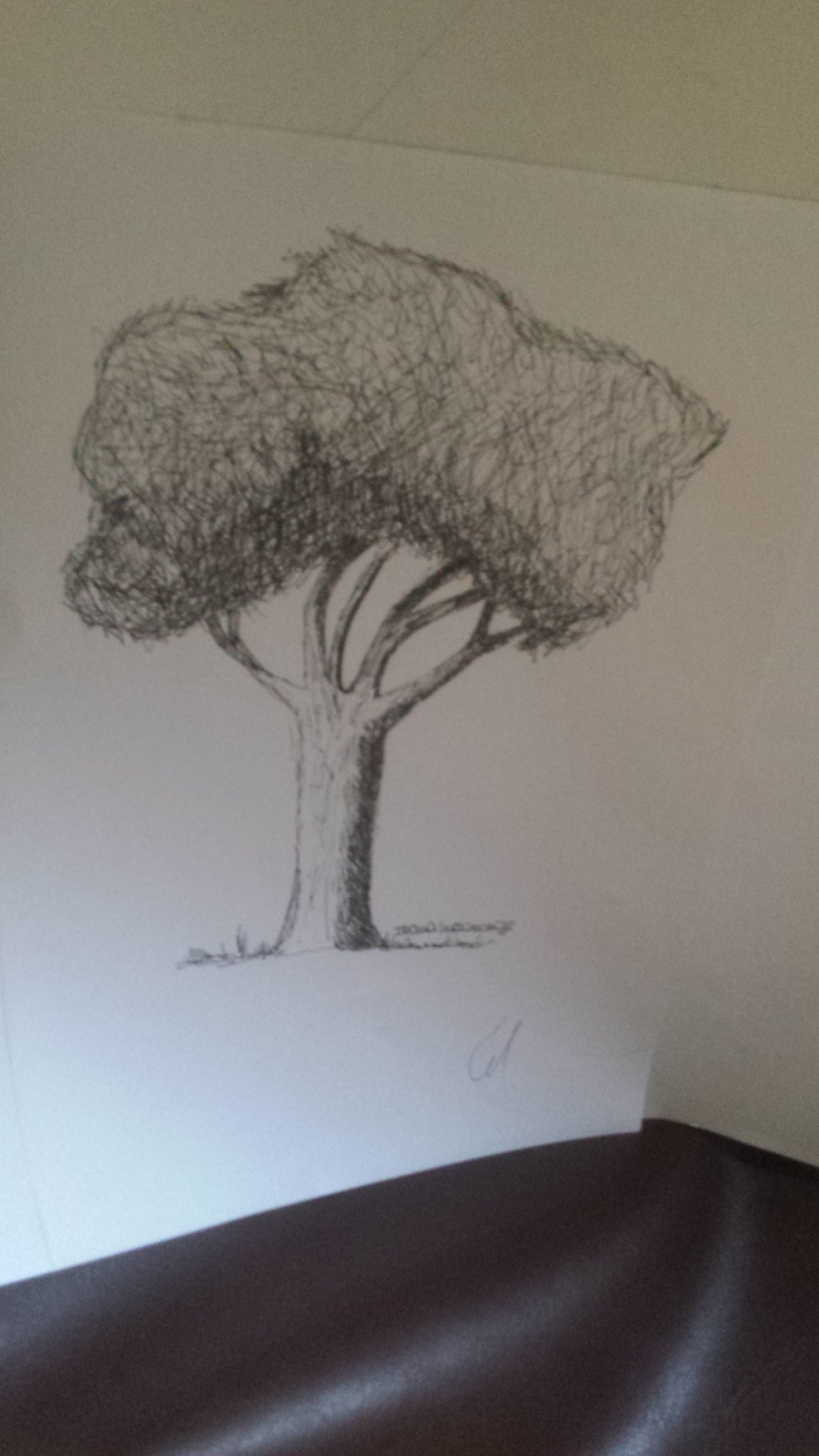This image showcases a pencil sketch of a tree rendered on a piece of horizontal paper, positioned at an angle such that the left side is elevated while the right side slopes downward. The tree depicted has a robust, wide base accompanied by a patch of grass on the left. On the right side of the paper, tiny, nearly imperceptible words are inscribed in pencil. The branches of the tree in the middle section slant toward the right, while those on the left curve gracefully to the left. The upper portion of the tree consists of extensive pencil shading, creating the effect of dense foliage without distinct leaves. Notably, the bottom right corner of the paper exhibits a small tear or cut. The sketch is set against a background that shows the paper resting on a white table at the top of the photo, and at the bottom, a black fabric can be seen.